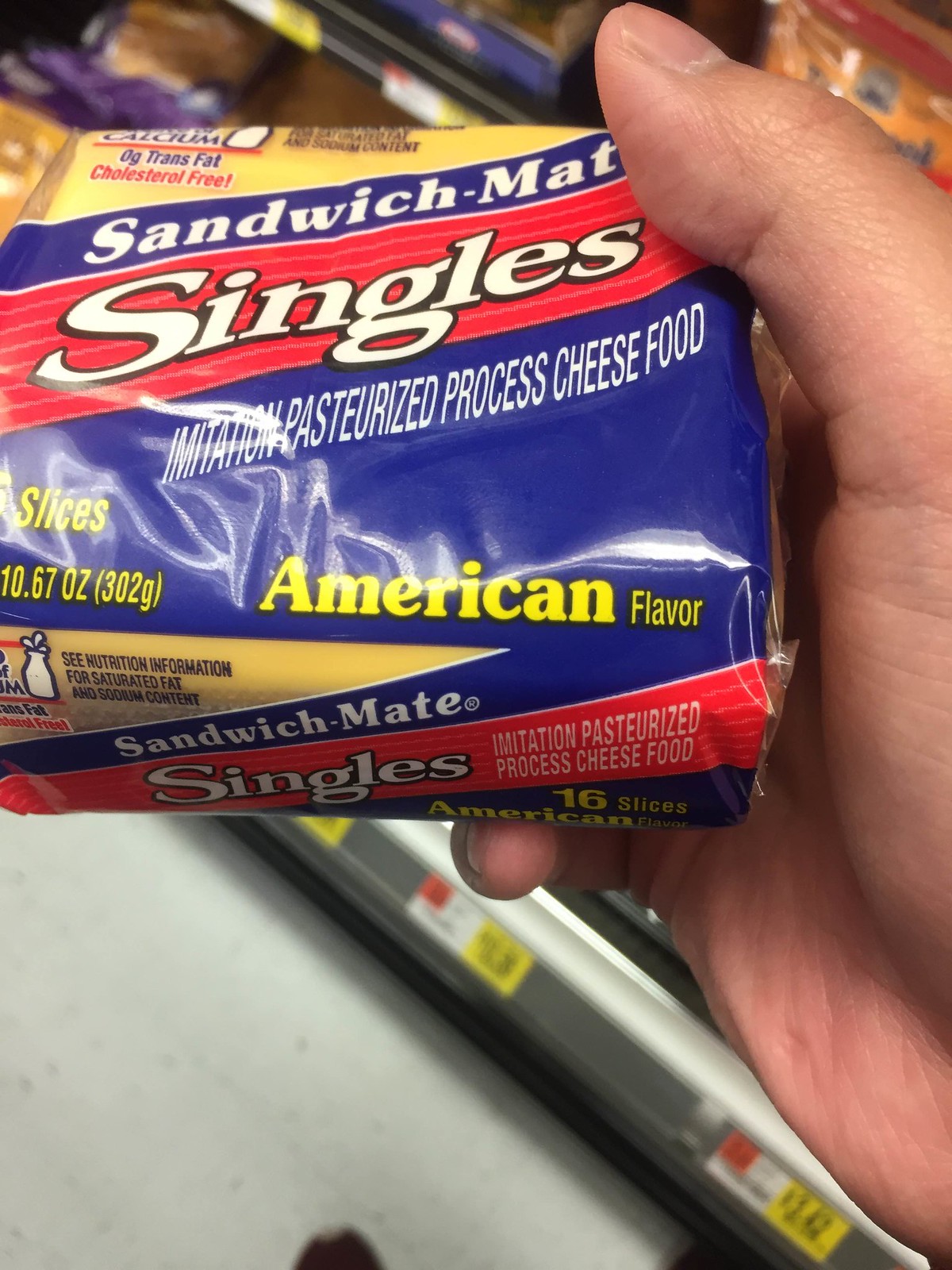In a close-up image taken in a grocery store, a reflective white floor forms the background where a person is standing. There's a bottom shelf visible behind them with a silver exterior adorned with price tags and stickers. Prominently displayed in the image is the person's right hand, holding a pre-packaged packet of cheese slices. The hand showcases the palm, thumb, and pinky finger gripping the product. The cheese packet is labeled "Sandwich Made Singles," indicating it contains 16 slices of imitation, pasteurized processed cheese food, described as American flavor. The individual cheese slices are yellow and individually wrapped, and the product is clearly meant for making sandwiches.